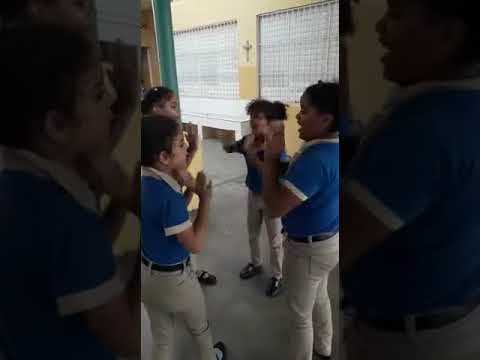In the image, four young girls are depicted standing in a circle in a brightly lit classroom, engaged in a clapping game. They are all dressed in matching uniforms consisting of blue t-shirts with white collars and trim on the sleeves, khaki pants held up by black belts, and black shoes. The girls, who have darker skin tones and black hair, appear lively and joyous, with their hands outstretched and faces animated as they participate in the game. The scene suggests a relaxed and collaborative atmosphere, possibly indicative of a private Catholic school, as evidenced by the cross on the yellow wall in the background. The classroom is softly lit by natural light streaming in through the windows, creating a warm and inviting environment.